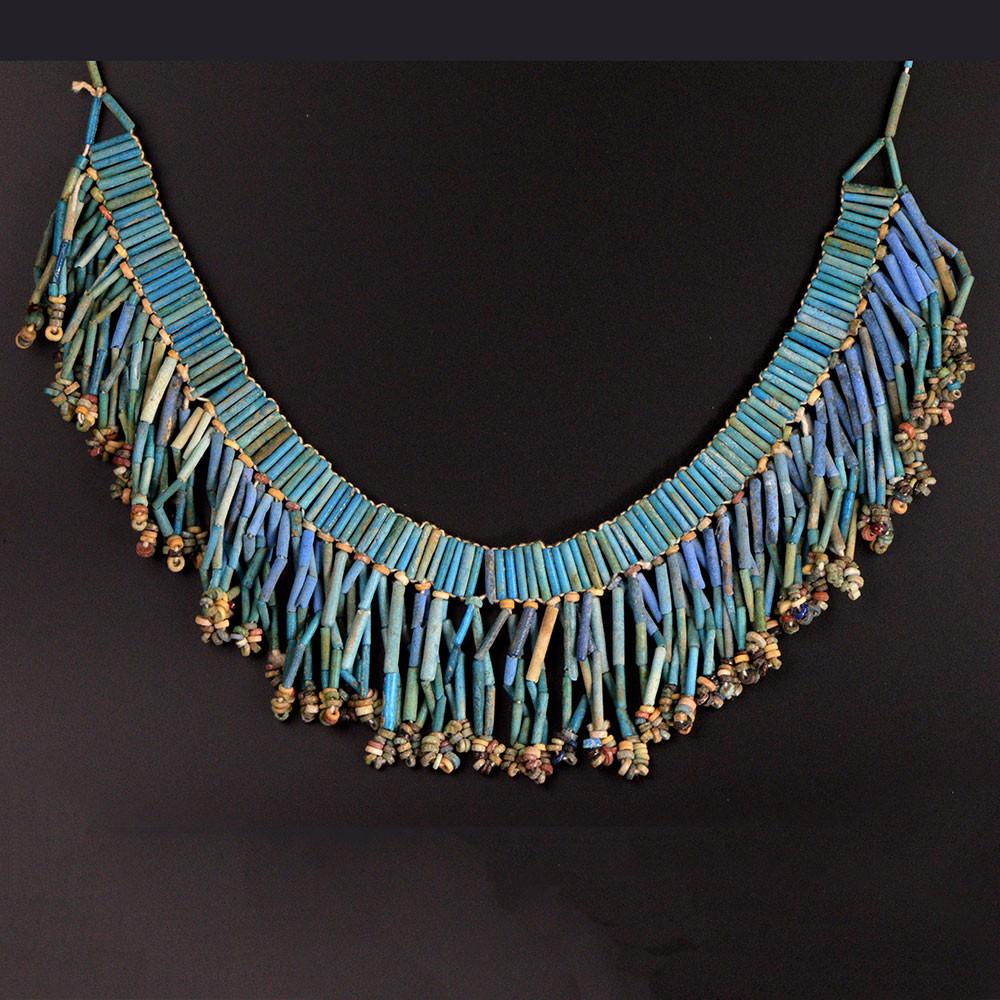The image showcases a large, U-shaped necklace, likely of tribal origin, possibly crafted by Native American artisans. The striking piece is displayed against a black background, suggesting either a museum exhibit or a professional setting to highlight its intricate design. The necklace comprises primarily vertical blue beads, interspersed with smaller seed beads in various colors such as yellows and tans, creating a visually engaging pattern. The composition also includes off-color greens, indicating that the beads are not uniformly matched. At the ends, the necklace features smaller circular beads in earthy tones like brown and orange. The central hanging beads, also blue, add to the elaborate and vintage aesthetic of this traditional piece.